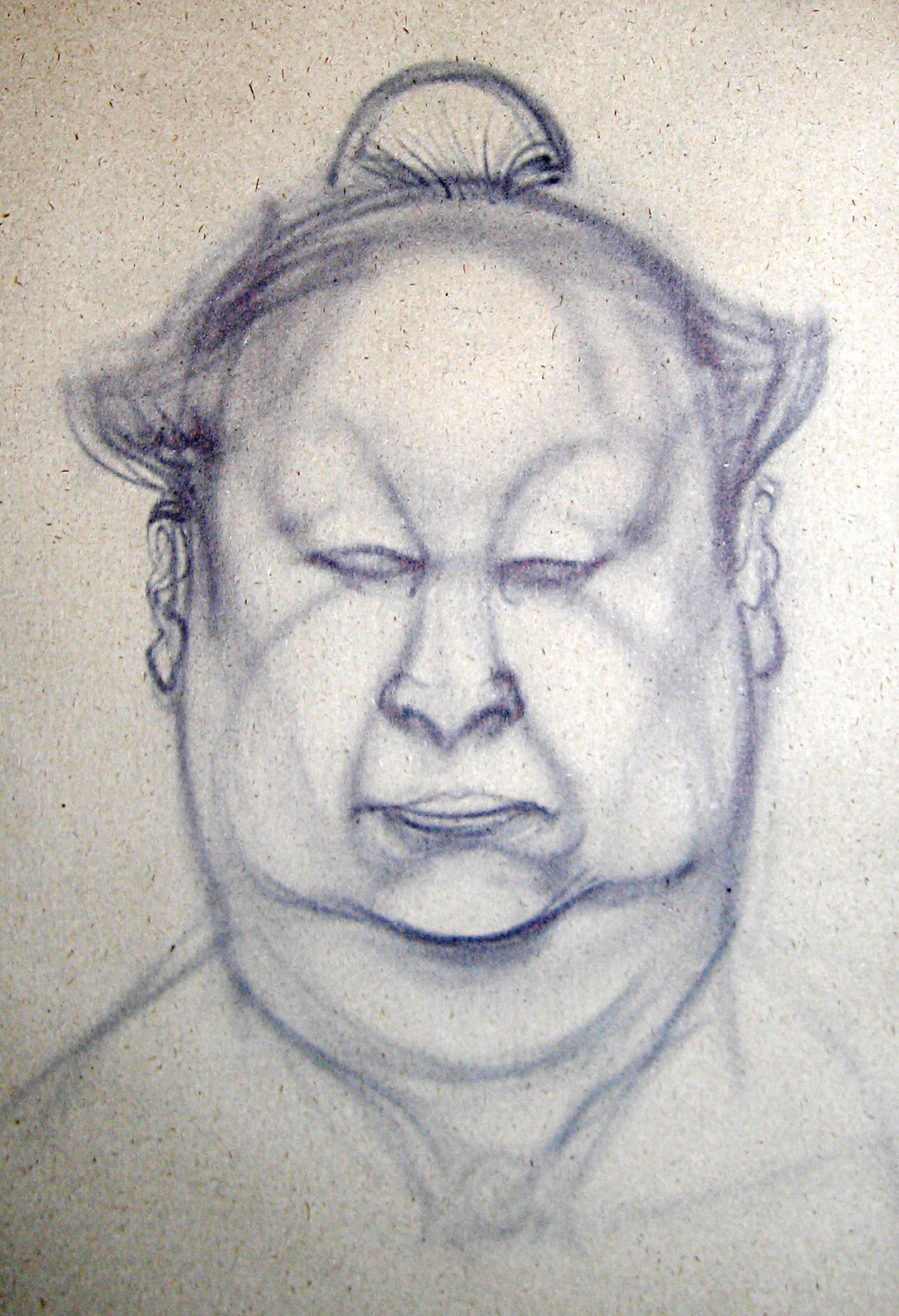This is a detailed drawing of an Asian man on recycled, speckled paper, characterized by small gray and brown flecks. Drawn in blue ink, the man features an oval face with slightly overweight proportions, wispy hair to the sides with almost no hair on top. He has narrow, small eyes, a wide nose, thin lips, and a double chin with excess skin beneath it. The man wears a small circular hat or object on his head, adorned with tiny lines connected to a bottom headband and wings fanning out above his ears. His neck and lightly sketched shoulders are visible, completing the portrait within the frame.